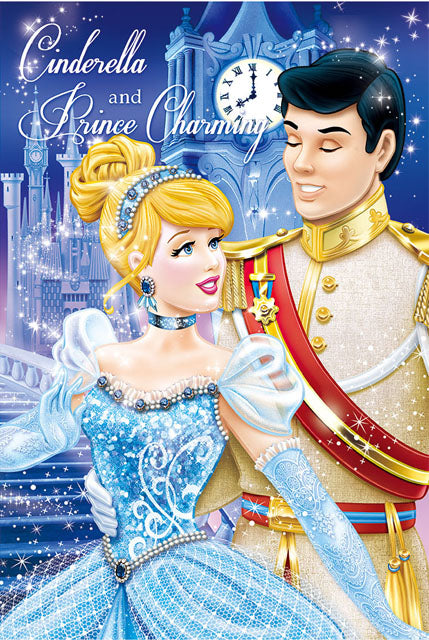The image is a vibrant movie poster for the cartoon 'Cinderella,' primarily featuring Cinderella and Prince Charming. Cinderella stands on the left, adorned in a stunning blue and white princess dress with puffed sleeves and ruffles. She wears elegant, long pastel blue gloves that reach from her elbows to her hands. Her blonde hair is styled with a blue gem-studded bandana, and she accessorizes with a matching blue choker around her neck. A bejeweled belt cinches her waist, adding a delicate sparkle to her attire.

To the right stands Prince Charming, who has dark hair and is dressed in an elaborate, gold-themed military uniform. His uniform features gold epaulets, a gold-collared jacket with gold buttons, and a belt with blue and red accents adorned with gold tassels. He wears a red sash emblazoned with several medals that drapes diagonally from his right shoulder to his left waist. Prince Charming gazes adoringly at Cinderella.

In the background, a majestic castle and a towering clock tower enhance the fairy-tale atmosphere, with the clock hands pointing to 8 o'clock. The sky is scattered with twinkling stars, completing the enchanting scene. The title 'Cinderella and Prince Charming' is prominently displayed in white lettering against a light blue backdrop in the upper left corner.